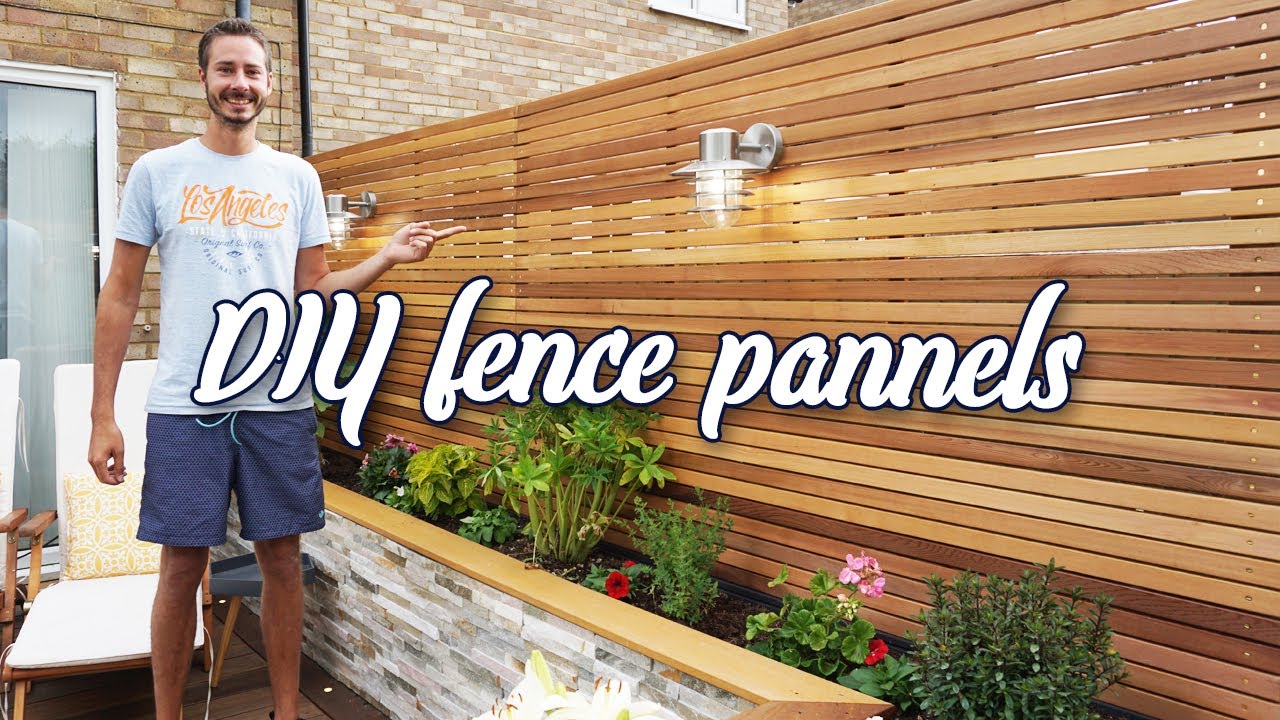In this wide horizontal photograph, a tall, lean man around 30 years old, clad in blue shorts and a white t-shirt emblazoned with "Los Angeles" in orange letters, smiles while pointing at a newly constructed wooden fence. The man, with brown hair and a beard, stands on a deck or patio area attached to a brick building, which also features two white lounge chairs and a sliding glass door in the background. The variegated medium wood-colored fence, which stands approximately 5 feet tall, has a sign with large white letters spelling "DIY Fence Panels" (notably misspelled as P-A-N-N-E-L-S). The fence, adorned with two vintage-style silver lights, is set within a planter filled with a variety of blooming plants and flowers, showcasing a stone facade. The setting and the gentleman's gesture at the fence suggest this is an advertisement promoting DIY fence construction.